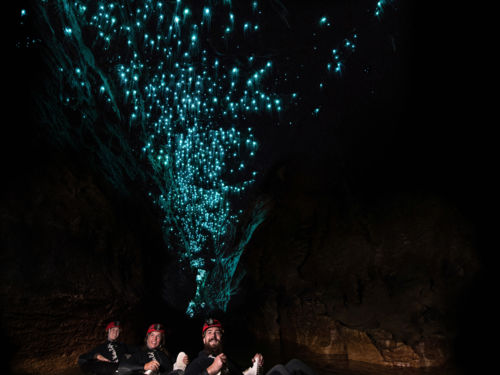The image depicts a scene inside a dark cave, where three individuals are huddled together, illuminated by their red hard hats, each equipped with a centered light. The trio includes a man on the right and two women on the left, who all appear to be engaged in writing or taking notes. Above them, an ethereal, shimmering display of light blue, almost turquoise, illumination spans the width of the image, creating a wave or tree-like formation. These lights, evocative of fireflies or some other form of bioluminescence, provide a stark contrast against the cave's enveloping darkness. The surroundings include dark rocks, and possibly water, adding to the mystique and allure of the subterranean environment. The overall scene captures a moment of scientific exploration and wonder amidst the cave's natural light show.